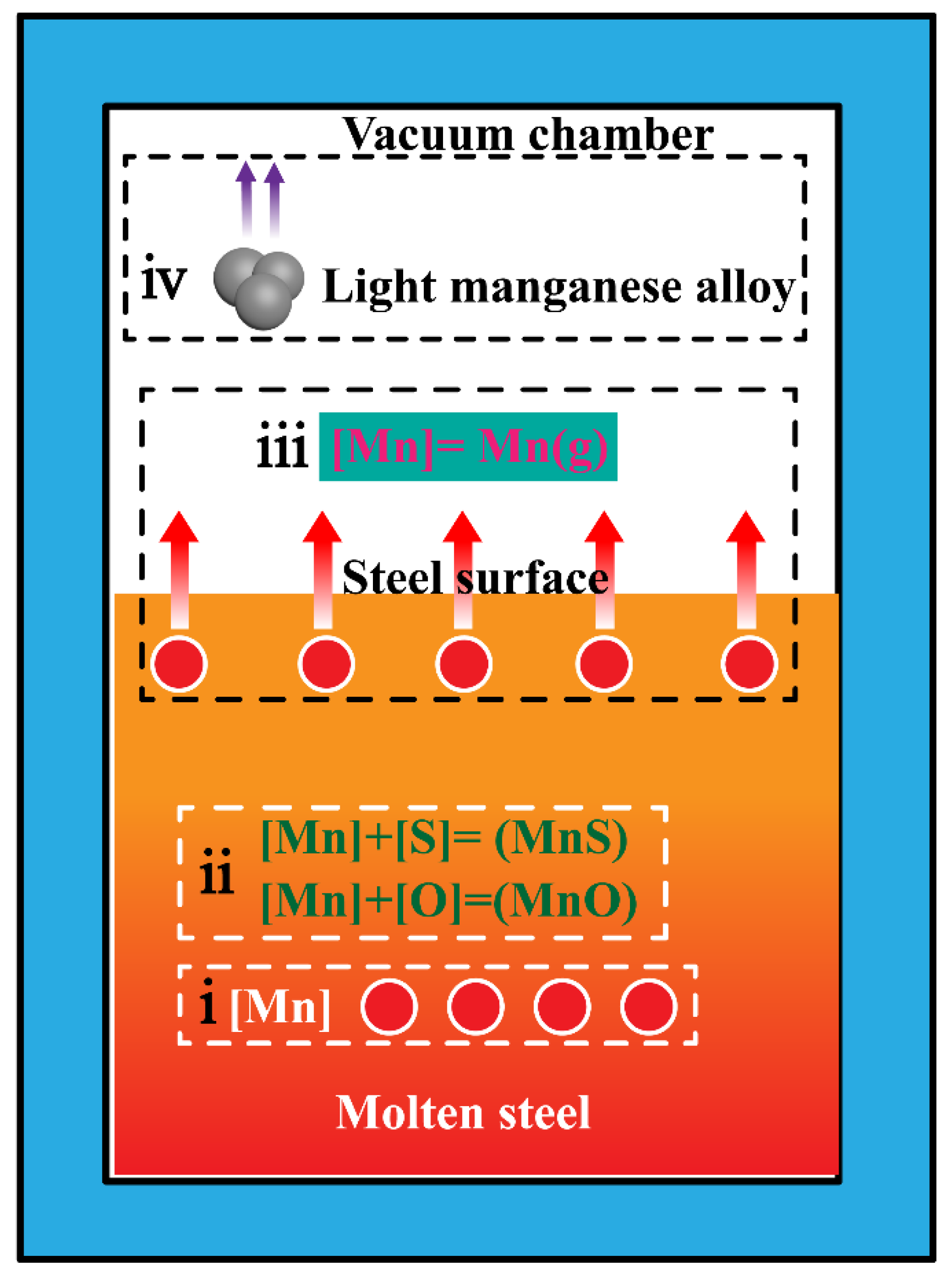This image is a detailed educational diagram, set within a rectangular format approximately 5 inches high and 4 inches wide, delineated by a thin black border with an inner lighter blue outline. The main content is housed within an inner rectangle also with a black outline.

The diagram's upper half features a white background with the bold black print title "Vacuum Chamber." Below this is a horizontally oriented dashed-line rectangle. On the left side of this rectangle, it displays "IV" in lowercase black print. To the right are three gray circles, bunched together with two purple arrows pointing upward, labeled "light manganese alloy."

Descending to the next section, there's another horizontal dashed rectangle, which is slightly taller. Its top center reads "III" in lowercase black print. This section has a greenish-blue rectangular background that features a bright pink print equation: "(Nn = Mn)G." Below this, set against a light orange background, are five dark orange circles with white outlines and arrows pointing upwards, labeled "steel surface."

The diagram’s lower portion transitions to a gradient from light to dark orange. Here, two more equations sit within white-dashed rectangles. The top equation is labeled "II" in black print, with green print equations reading "Mn + S = MnS" and "Mn + O = MnO." Below this is another dashed rectangle, marked with a black "I," which includes "Mn" in white print alongside four orange circles with white outlines. At the very bottom of the diagram, in white print against the darker orange gradient, it reads "molten steel."